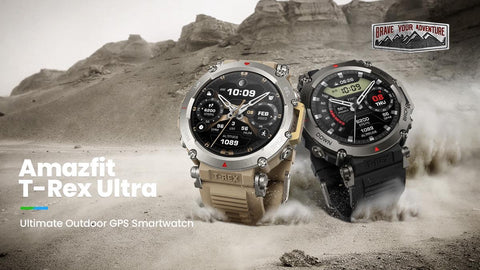The image is an advertisement for the AMAZEFIT T-REX ULTRA Ultimate Outdoor GPS Smartwatch, presented in a landscape format. The rugged background features a gray mountain with a triangular patch of sky in the top left, under a cloudy, gray sky, and a dusty, rocky terrain below. The highlight of the image is two robust, men's smartwatches displayed on the right, seemingly in dynamic motion, kicking up dust behind them. Both watches feature black faces with silver hands and multiple functions, displaying the time as 10:09. The watch on the left has a cream-colored band and a frame accented with brass-like elements, while the right-hand watch has a black band and a gunmetal frame. To the left of the watches appears the product name "AMAZEFIT T-REX ULTRA" in bold white text, with "ULTIMATE OUTDOOR GPS SMARTWATCH" beneath in smaller white letters. In the upper right corner, a logo in silver, red, and black, with the phrase "BRAVE YOUR ADVENTURE" in red text, adds to the adventurous theme. The scene is devoid of people, focusing solely on the durable watches and their rugged, outdoor setting.